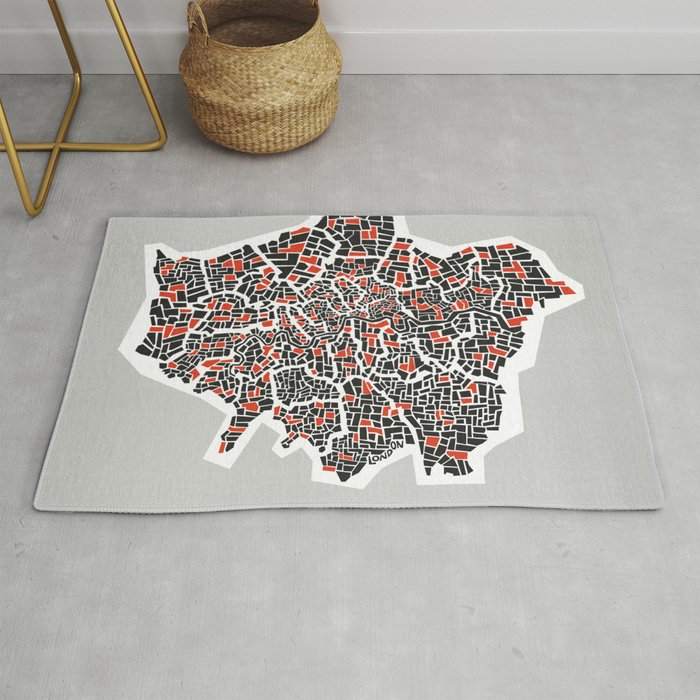This indoor photograph captures a gray floor, possibly made of concrete or a laminated material. At the center, there is an intriguing rectangular floor mat that appears to be a work of art. The mat is also gray and features an intricate design resembling a stylized map of London. The map is inset with a white border and depicts various blocks and arteries, akin to a mosaic. The blocks are rendered in black, white, and orange, creating a dynamic, amoeba-like pattern that represents different neighborhoods or sections of the city. The word "London" is inscribed at the bottom of the mat, confirming its thematic inspiration.

In the upper left corner of the photograph, there are brass-colored rods forming an X, likely the base of an unseen table. Slightly left of the mat's center, a wicker basket in light brown adds a touch of organic texture to the scene. A light gray baseboard molding runs along the top edge, meeting the light gray painted wall. The overall composition suggests a carefully curated space that blends modern artistic elements with functional objects.